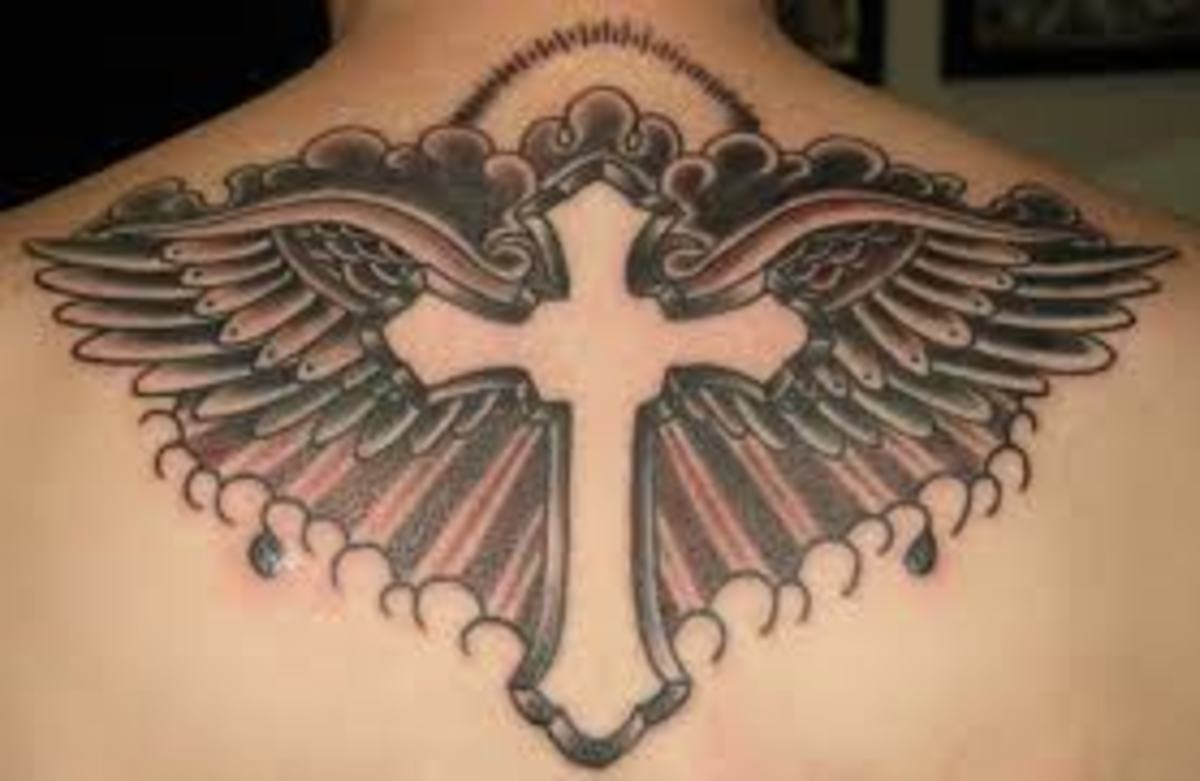In this color photograph of an apparently white male's upper back, the image is dominated by an intricately detailed tattoo spanning the base of the neck to the upper back, across the shoulder blades, and into the center of the back. The tattoo features a prominent, stylish cross at its core, outlined in white with the inner portion left as bare skin. Radiating from the cross are expansive wings, intricately shaded in black and red, evoking the image of an angel spreading its wings. The upper sections of the design incorporate cloud patterns, with radiant light emanating from the top. Below the wings, rays of sunlight extend downwards, accompanied by fine details resembling small heads or sun-like motifs. The backdrop of the portrait, slightly visible at the bottom of the frame, offers partial glimpses of other portraits, though the tattoo is unquestionably the focal point of the image.